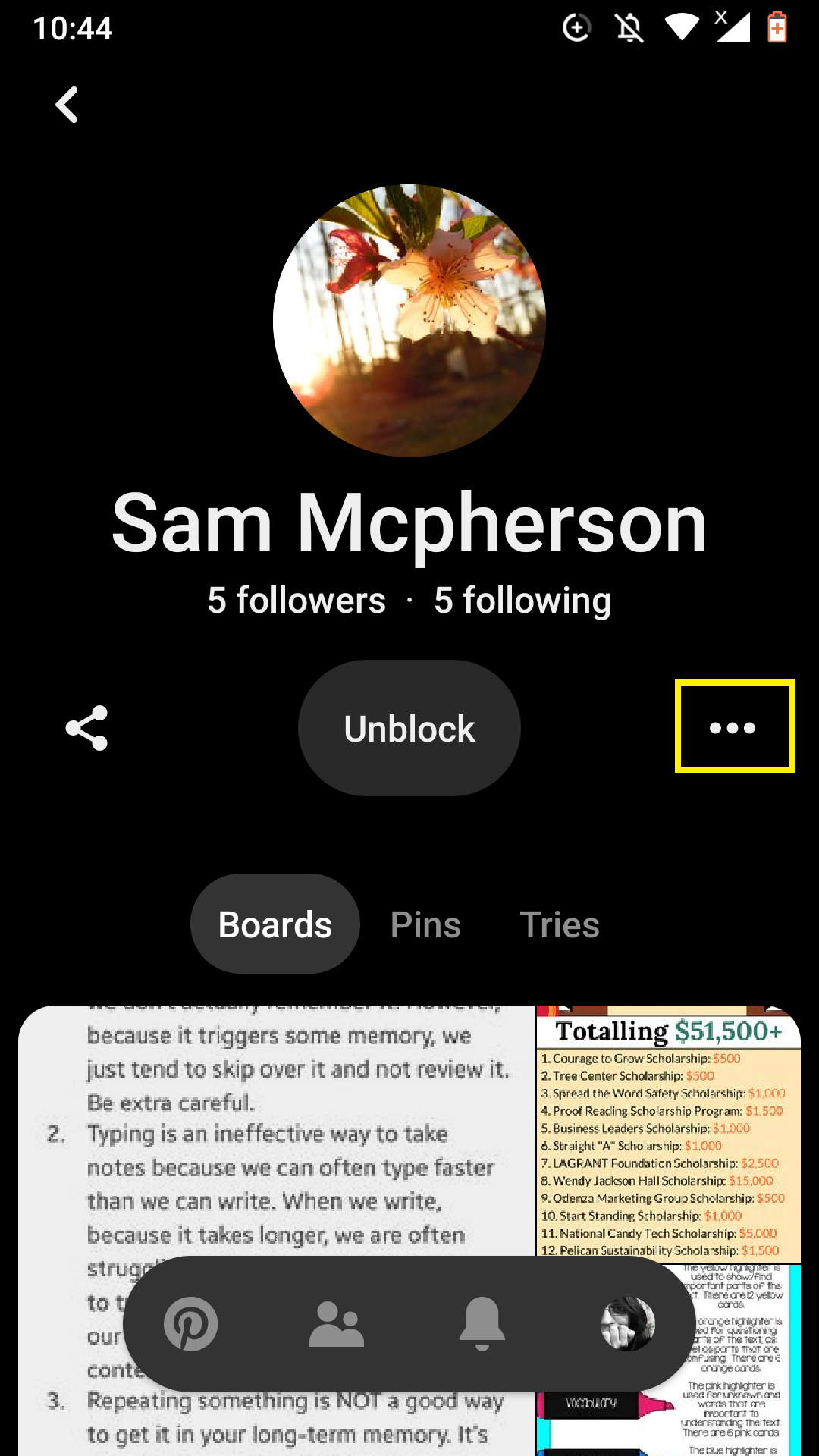This image is a screenshot of a Pinterest profile viewed on a cell phone. The phone's display is vertically oriented with a black background. At the top left corner, the time "10:44" is shown in white text. On the right side of the screen, there are several status icons: a bell with a line through it indicating the phone ringer is off, an upside-down triangle representing internet connectivity, a symbol showing no phone signal or data signal, and a battery icon.

In the middle of the screen, there is a circular profile picture depicting a white orchid with pink accents and green leaves set against a natural background that features indistinct elements of the ground, a hill, trees, and a bit of the sky. Below the profile picture, the username "Sam McPherson" is displayed in white letters, followed by "5 followers" and "5 following."

To the left below the profile details, there's a sharing icon. In the center, there is a button labeled "Unblock," and to the right, there are three horizontal dots enclosed in a yellow square. Beneath these elements, three centered buttons read "Boards," "Pins," and "Tries."

Further down the screen, a square area with white background contains text, and at the bottom, there is a navigation bar with several icons: the Pinterest symbol, a symbol representing people, a bell symbol, and a small round circle containing another profile image.